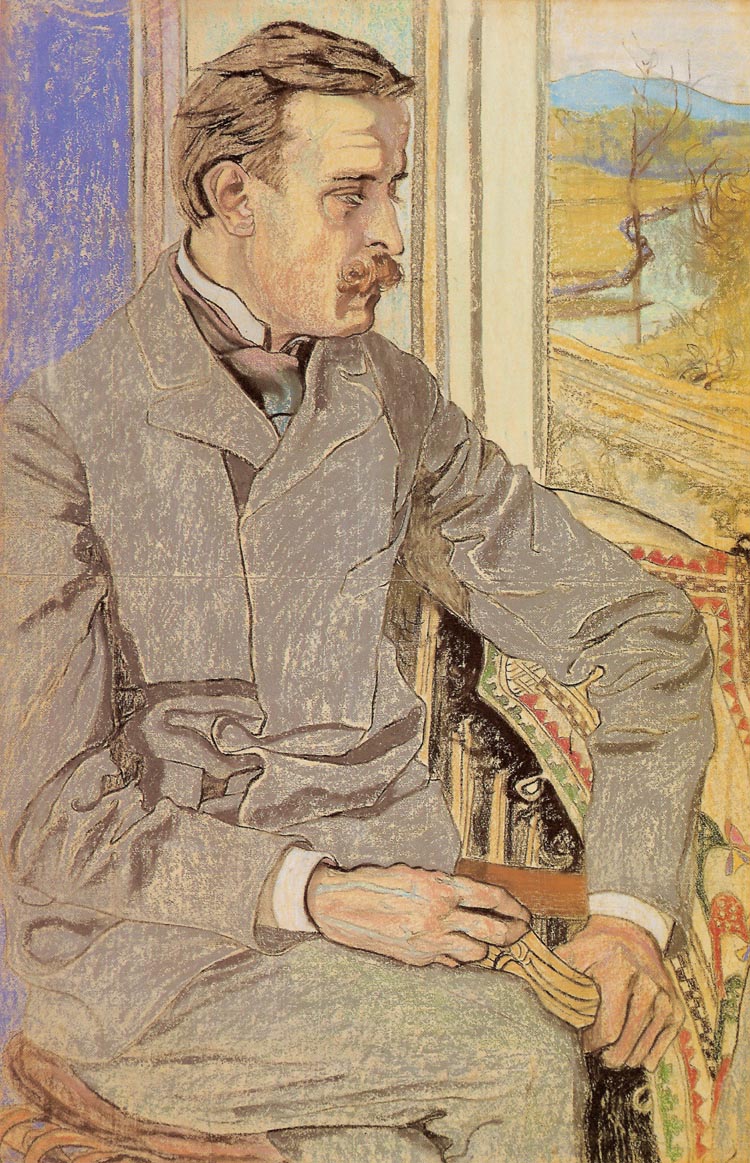This vertically aligned painting features a solemn man, appearing to be in his 40s, seated in an ornate, colorful chair. The man, depicted in a sketched style, sports a feathered brown hairstyle and a mustache. He is dressed in a gray suit jacket with visible white shirt cuffs and a tie. His right leg is crossed over his left, with only the upper portions of his legs visible. The man gazes contemplatively out a white-framed window to his right. Beyond the window, a narrow stream curves between two grassy banks, flanked by bare trees, with a hint of blue sky and a distant mountain. The background of the room appears to be painted blue, possibly incorporating elements of a second artwork. He holds an unidentified object, possibly a handkerchief, in his hand, adding to his introspective demeanor.